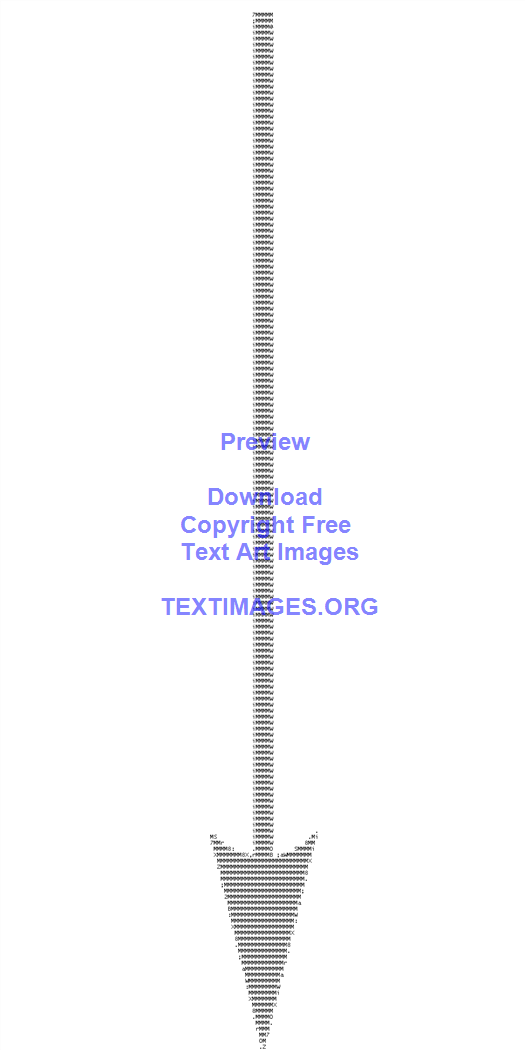The image features a downward-pointing arrow with a pixelated, gray appearance against a white background. The arrow's design includes a sharp tip and flat end, with an arched top leading to a long shaft. Superimposed on the arrow in light purple text are the words "Preview," "Download," "Copyright-free," "Text Art," and "Images," with the last line reading "TextImages.org." The overall style is reminiscent of simplistic, text-based art.